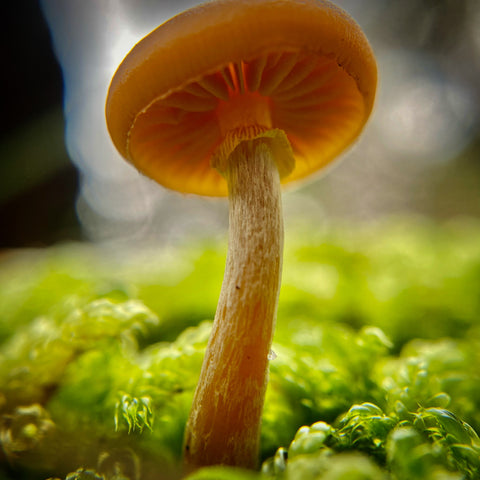The image is a detailed close-up of a small mushroom, approximately an inch tall, centered prominently within the frame. The mushroom features a smooth, round cap with a brownish-orange hue, reminiscent of an orange sliced in half, showing a distinct radial pattern of white spokes on its underside. The stem, textured in a light brown and pinkish tint, grows slightly askew to the left. It is emerging from a green, mossy, bumpy substrate. The photograph is taken from a low vantage point, capturing the gills or flutes underneath the cap. The background is softly blurred, with hints of green grass and vague white shapes, emphasizing the mushroom's details against the outdoor setting.